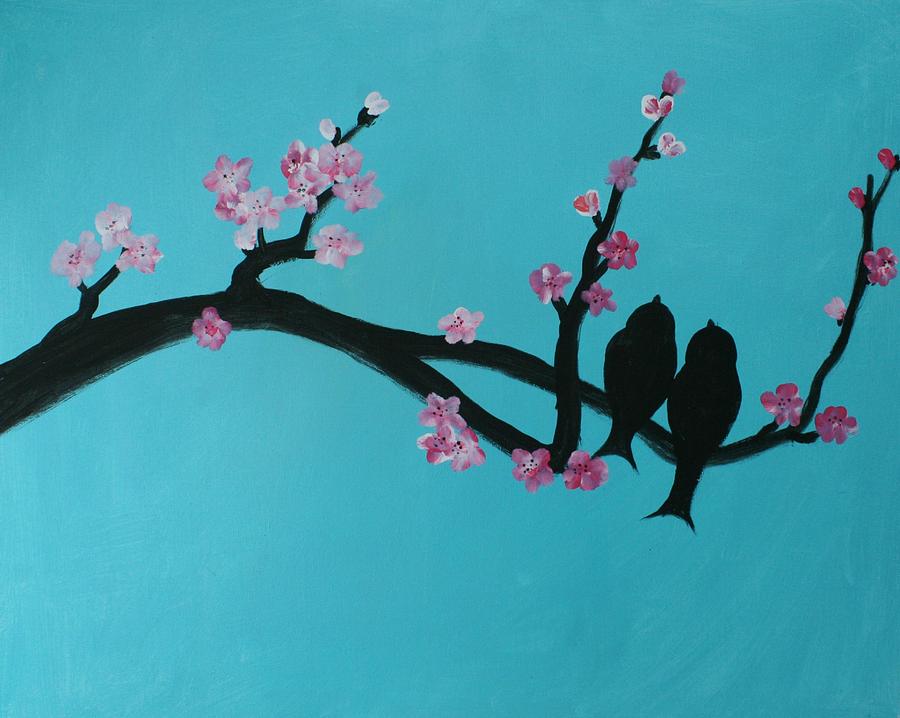This image features a piece of Japanese or Asian-inspired art set against a light blue, almost turquoise background reminiscent of a clear Carolina sky. Dominating the scene are intricate black branches, adorned with delicate cherry blossoms in various shades of pink, white, and darker mauve. The flowers cluster at the tips of the branches, revealing a mix of buds and fully bloomed petals. Two small silhouettes of birds perch on the branches, their distinctive curved tails and bifurcated feathers adding a whimsical touch. These birds are positioned to appear as if they are looking upwards, their beaks slightly tilted, completing the serene and enchanting tableau. The entire composition captures the elegance of nature with detailed brushstrokes, particularly noticeable in the curvature and texture of the branches.